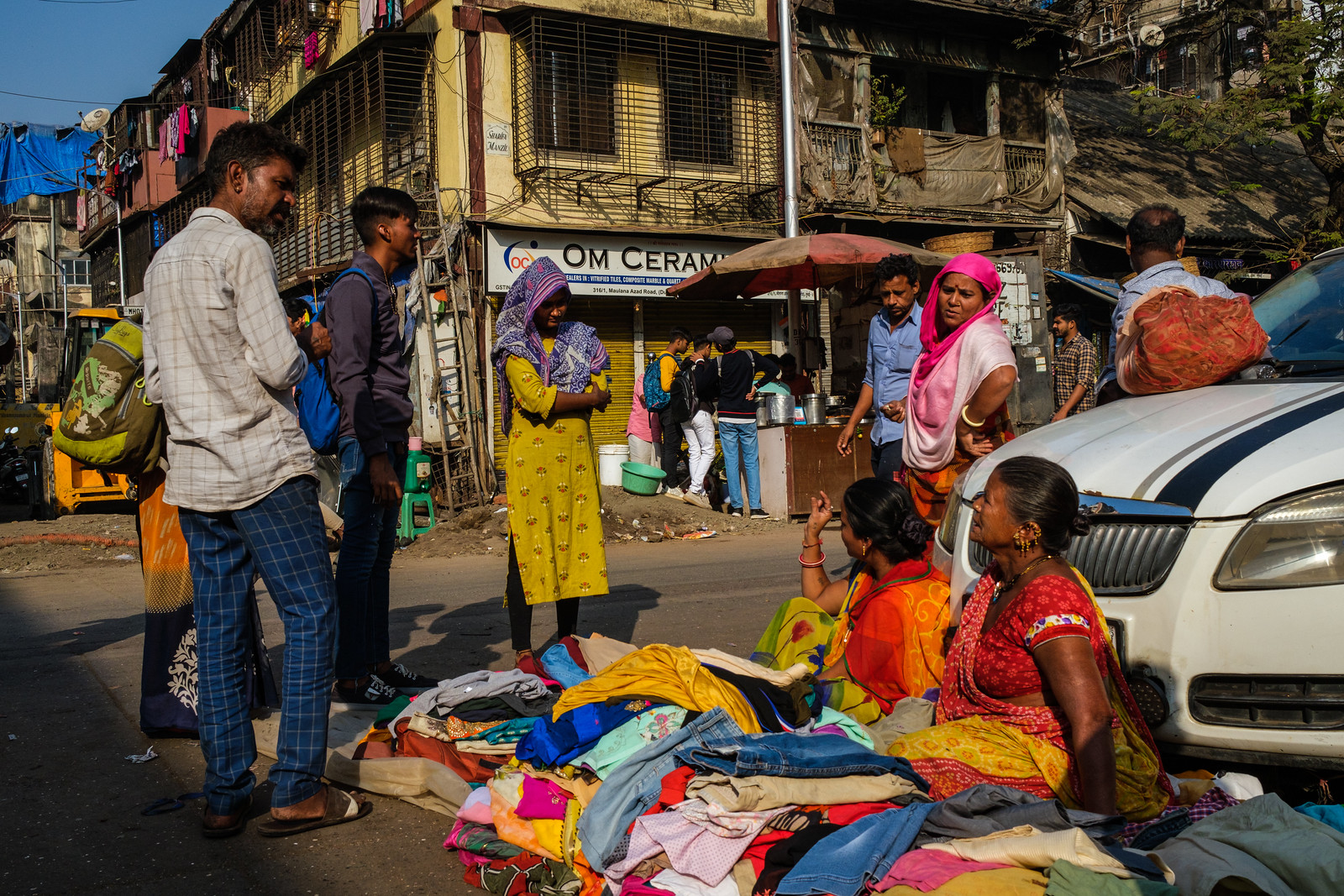The image depicts a scene from a poor neighborhood, possibly in a third-world country, characterized by its rundown buildings and decrepit surroundings. In the foreground, two women are seated on the ground, leaning against a white car with a blue stripe. A large pile of colorful clothing, including jeans, shirts, blouses, and dresses, is spread out in front of them, suggesting that they might be selling these items. Surrounding the women are several people engaged in various activities: two men with distinct outfits—one in blue pants and a white shirt, the other in black pants and a purple shirt—stand to one side, while a few other men and women converse nearby. In the background, more individuals, including children, gather around what appears to be a food stand with a faded umbrella. The buildings, painted in muted yellows, reds, and browns, feature barred windows and clothes hanging out to dry, further emphasizing the area's impoverished state. Despite the bleak environment, the people's clothing adds a splash of color to the scene, with vibrant yellows, reds, and greens standing out against the dusty backdrop.